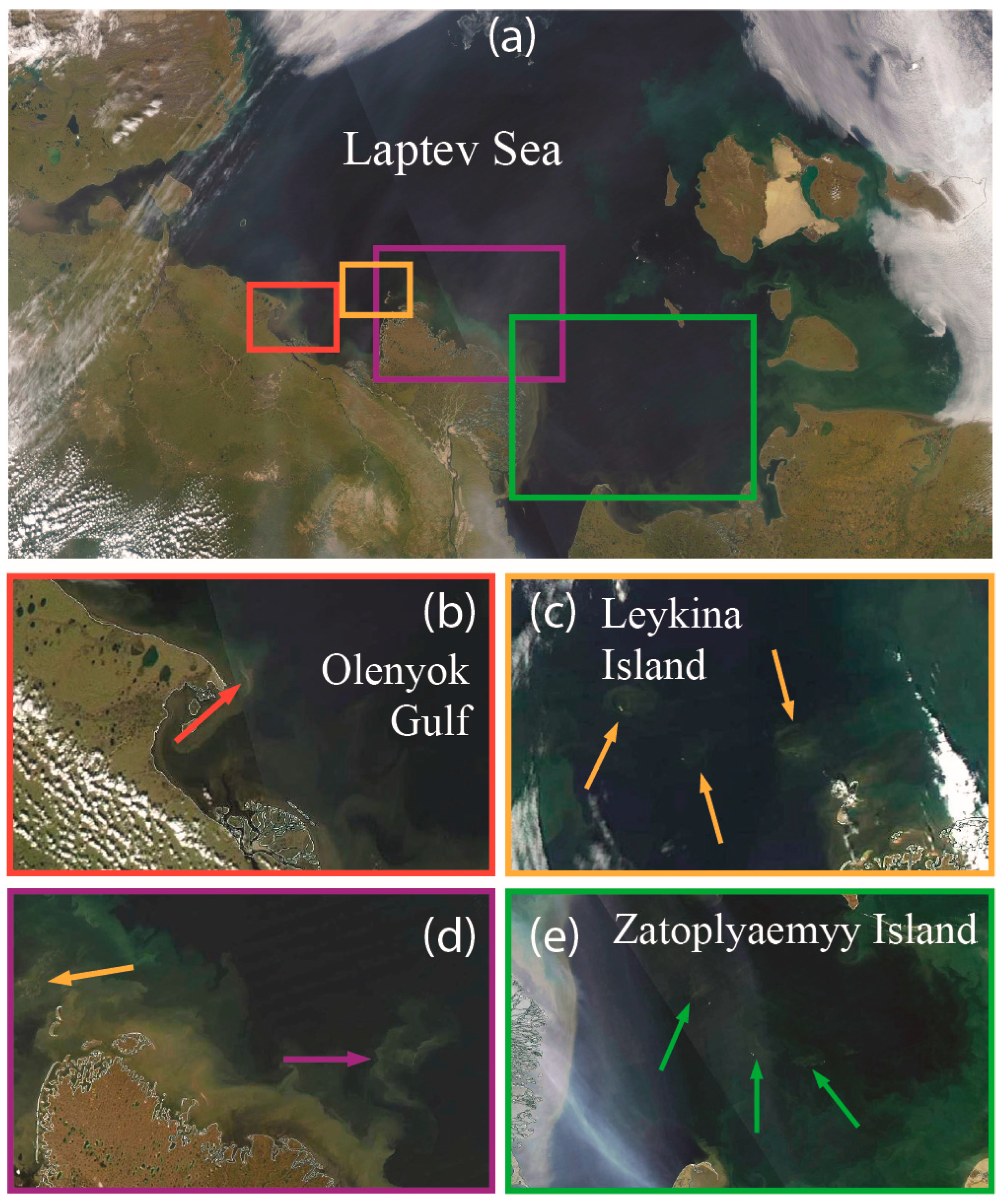In the image, we see a series of panels, with the top half dominated by a large, horizontal satellite view featuring the Laptev Sea. The sea is depicted in shades of greenish-blue, bordered by brown and green landmasses, and some cloud cover is visible. Overlaid text in the center reads "LAPTEV-C". Superimposed on this main image are four colored rectangles—green, orange, yellow, and purple—each marking specific areas.

The green rectangle spans from about a third of the way over to the center from the right, while an orange rectangle is slightly off-center and smaller than the green rectangle. A smaller, reddish rectangle is noted near the center, with a pinkish rectangle occupying the top corner adjacent to it. A darker orange rectangle lies next to this pinkish section.

Below the main image, four specific panels detail the marked areas from the top image. The orange panel corresponds to the Olenjak Gulf, a mix of land and water. The yellow panel highlights regions to the left and right of the landmass. The purple panel designates Zato Plissimi Island, with green arrows indicating its location on the larger map. Finally, the bottom left panel identifies Lake Kena Island, with accompanying orange arrows pointing to relevant spots on the upper map.

Overall, the image intricately outlines sections of the Laptev Sea and its various geographical features, providing a detailed high-altitude perspective that might be captured by a satellite.